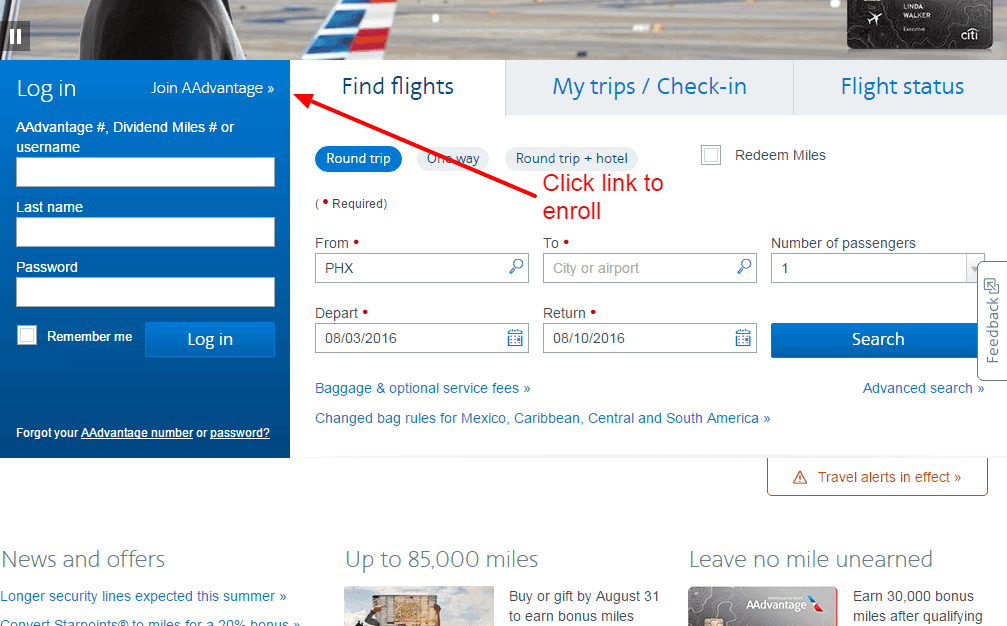The image depicts a flights booking page. On the left side, there is a login section with fields for 'AAdvantage Number or Username', 'Last Name', and 'Password'. The 'Remember Me' option is unchecked, and a 'Login' button is present. Below the login fields, there is a link for users who have forgotten their AAdvantage number or password. 

The page also features various navigation options including 'Find Flights,' 'My Trips,' 'Check-In,' and 'Flight Status.' Options for booking 'Round Trip,' 'One Way,' 'Round Trip + Hotel,' and redeeming miles are available. The fields are pre-filled with 'From: Phoenix' and there is a clickable link for new users to enroll in the AAdvantage program, highlighted by an arrow pointing towards 'Join AAdvantage,' accompanied by a note stating 'Click link to enroll.'

Further down, there’s a 'News and Offers' section. Headlines in this area include warnings about longer security lines expected over the summer, and a promotion offering up to 85,000 bonus miles for buying or keeping miles by August 31st, with the slogan 'Leave No Mile Unearned.'

The color scheme includes blue, orange, and black, set against a white background, contributing to a clean and professional appearance.